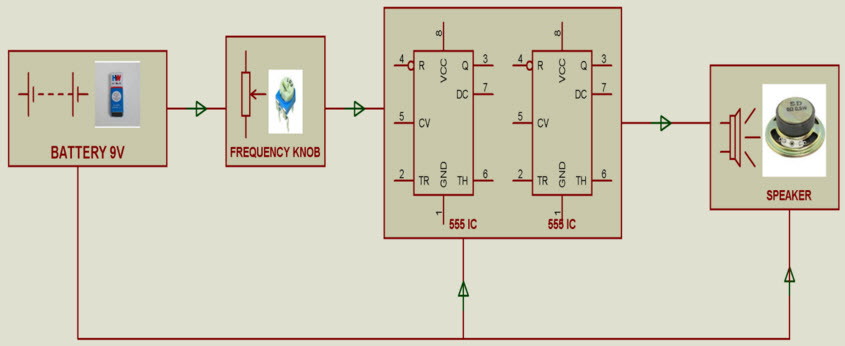This image is a detailed schematic of an electrical circuit set against a light gray-green background. The diagram uses red lines and boxes to outline the circuit components, with prominent green arrows indicating the flow of electrical current.

On the far left, there's a red-outlined box labeled "Battery 9V," containing a white square with an illustrative picture of the battery. Connecting to the right, a red line is interrupted by a green arrow, leading to another red box labeled "Frequency Knob." Inside this box is a white rectangle with a blue and green drawing, signifying the frequency knob component.

Continuing rightward, another red line, also interrupted by a green arrow, leads to a larger red-outlined box labeled "555IC." This box contains two smaller rectangles with black numbers and letters inside, indicating specific electrical values or connections.

The circuit then connects via another red line and green arrow to a final red box on the far right, labeled "Speaker." Inside this box are a few lines and rectangles, one of which is angled at the top, and a white rectangle containing a green illustration representing the speaker.

Additionally, a red line runs from the "Battery 9V" box directly to the "Speaker" box, and another line branches off to connect to the "555IC" box, ensuring power distribution to all components. The interconnected lines facilitate the complete circuit, visually represented with clear directional arrows guiding the current flow between the battery, frequency knob, 555IC, and speaker.